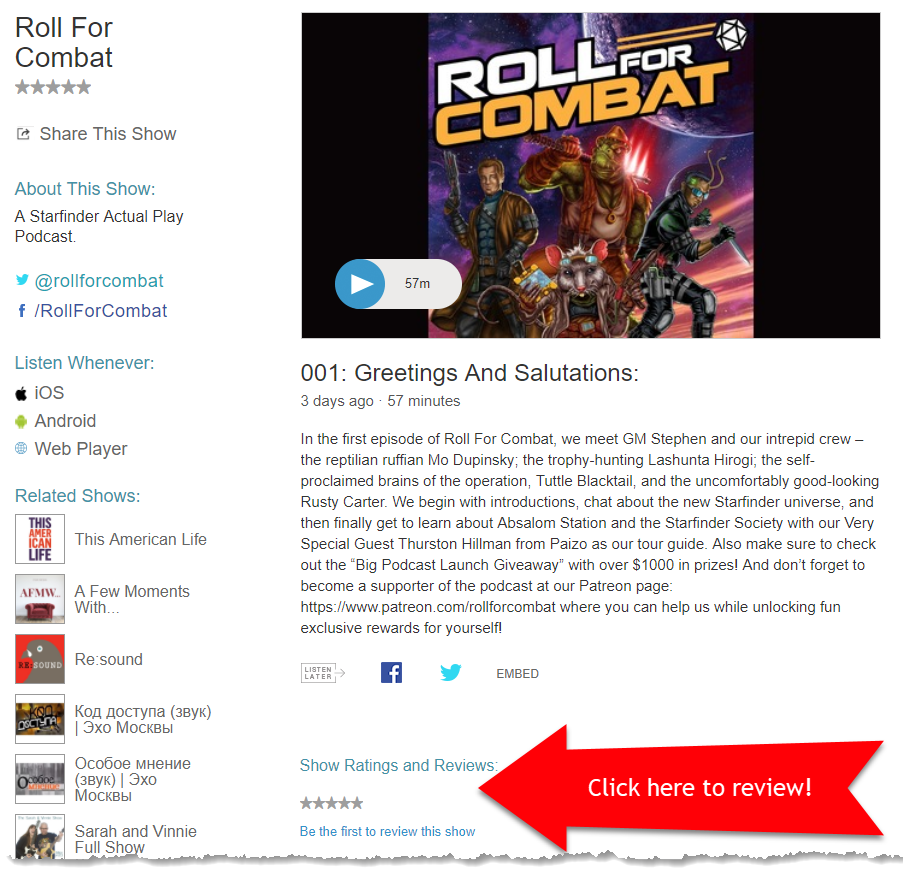The screenshot displays detailed information about a show titled "Roll for Combat." On the left-hand side, there's a vertical menu bar which includes the show's title at the top followed by gray star icons that allow users to rate the show. Below this, options to share the show on various social media platforms are provided alongside the social media handles specific to the show. There are also links where users can listen or watch the show on iOS, Android, or a web player. Additionally, a section lists related shows such as "This American Life," "A Few Moments With," "Resound," as well as some shows in Russian.

To the right of this menu bar, a large thumbnail image of the show's title cover poster is displayed with an overlaid play button, indicating that the show is 57 minutes long. Beneath this image, more specific details about the show are presented, including information about episode one titled "Greetings and Salutations." A brief synopsis of the episode is also provided.

Further down, there is another mention of social media handles followed by a "Show Ratings and Reviews" section. Here, gray stars are again displayed for users to click and rate the show. A prompt encourages users to "be the first to review the show," accompanied by a prominent red arrow pointing at the gray stars with a message directing users to "click here to review." The layout clearly indicates where viewers should go to provide their ratings and reviews.